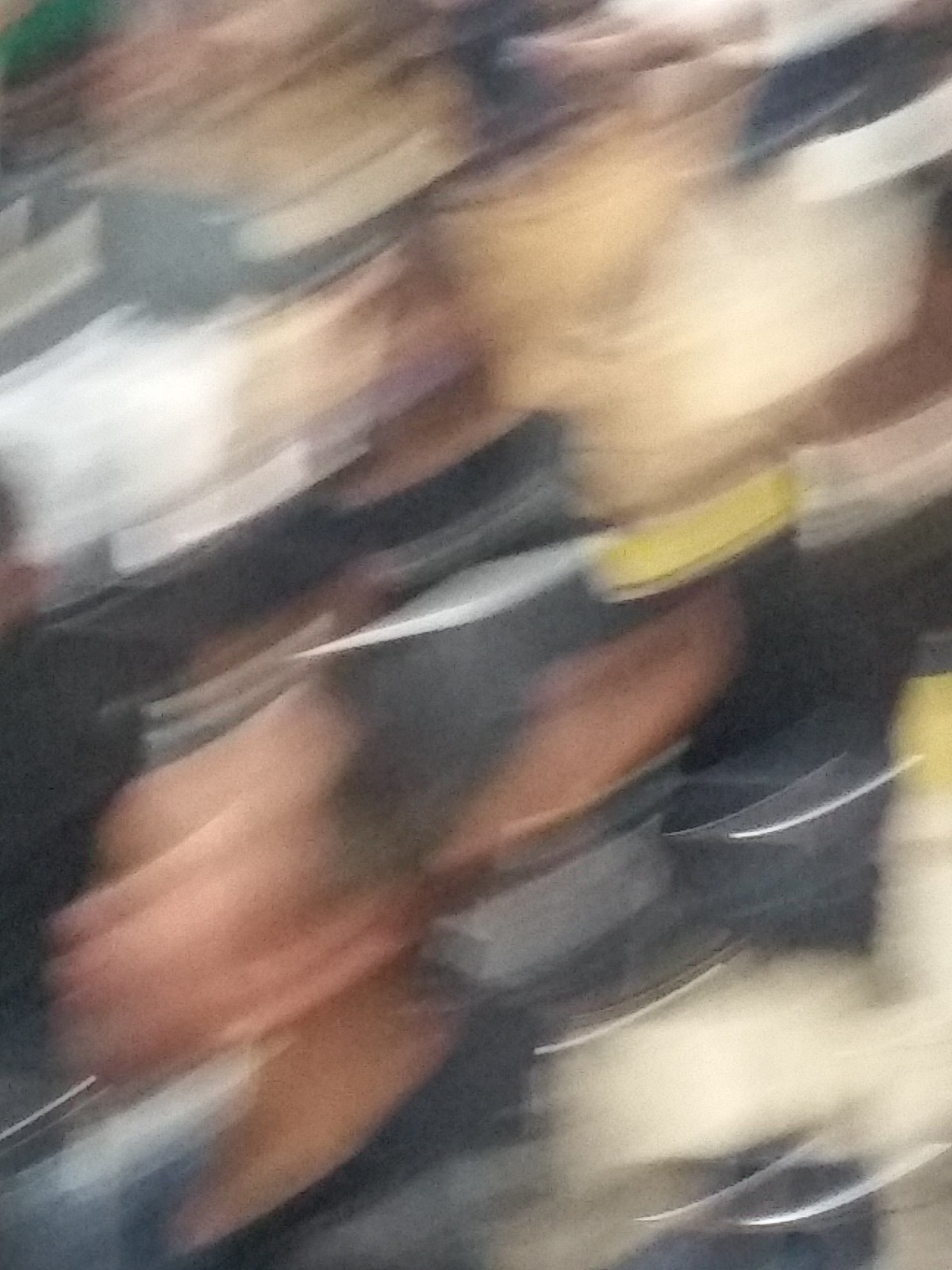An indoor color photograph captures a heavily blurred image, seemingly due to camera movement. The colors sweep from the lower left to the upper right at an approximate 30 to 45-degree angle, creating a pattern of streaks and splotches. In the lower right, we observe some white hues, while the foreground predominantly displays shades of blue. Towards the center and the left, vivid orange, yellow, and white streaks mix with occasional dashes of pink. Additionally, the upper right corner features more white splotches. The blurred elements suggest they could be items on a supermarket shelf, possibly with white labeling, though nothing is clearly identifiable. The image, taken indoors, is grainy and lacks any discernible text or print, giving it an abstract, almost geometric composition composed of streaked colors and splotches.